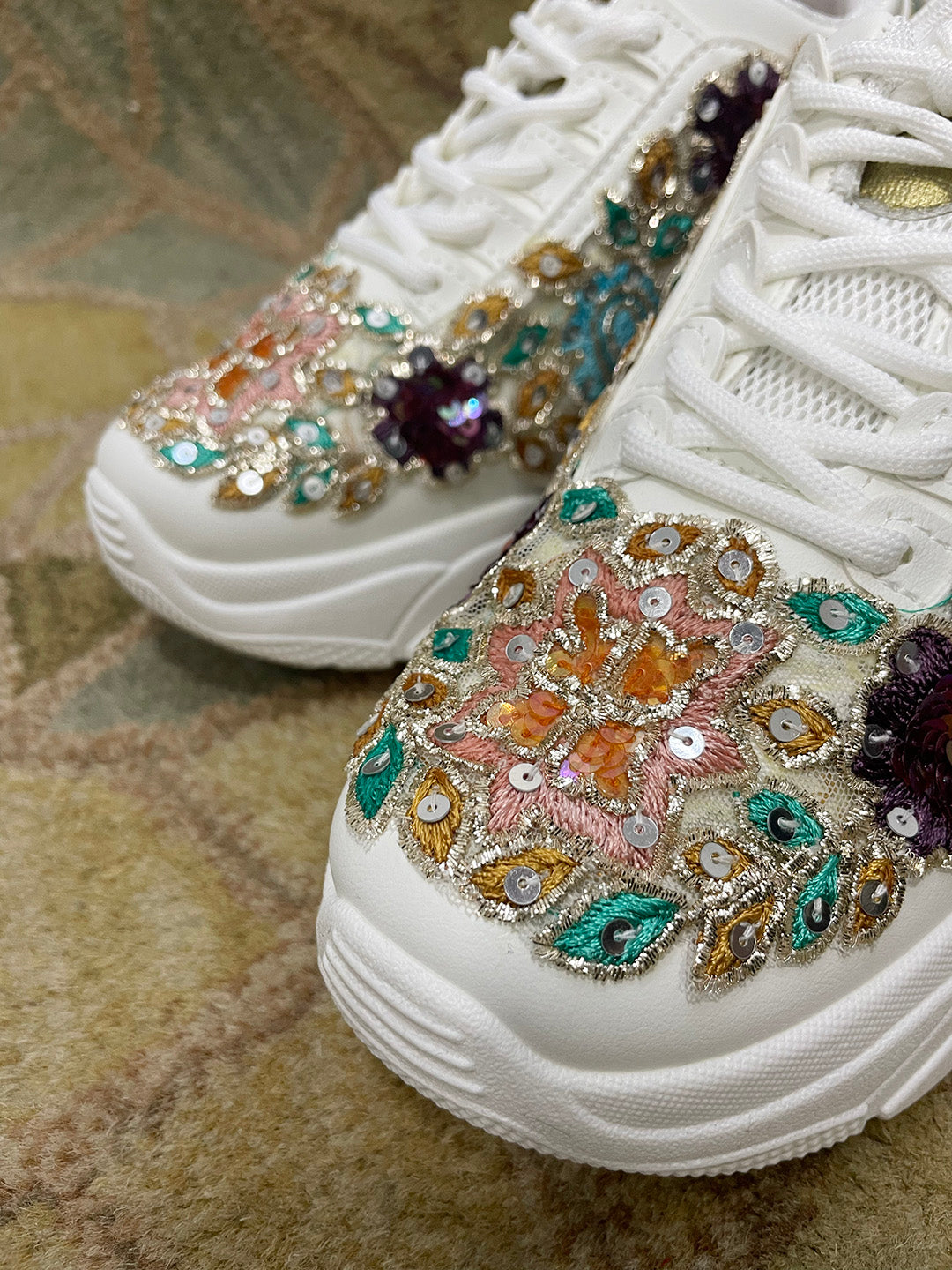This is a close-up vertical image of a pair of white tennis shoes set against a brownish background that resembles a carpet. The shoes, angled diagonally from the upper right-hand corner down to the center-left of the image, display intricate details. Dominating the design are elaborate patches in the shape of leaves, adorned with small silver sequins and rhinestones that reflect light when it strikes them, creating a glistening effect. These patches feature various colors, including turquoise, orange, gold, pink, and brown. On the front of each shoe, prominently placed patches form flowers and leaf shapes, with the flower designs made using pink and orange threads. The shoes have white laces running up to the point where they exit the image's frame. You can also see partial views of both sneakers, primarily focusing on the toe area and the sides adorned with these intricate, colorful embellishments. The background shows glimpses of a tan and gray carpeted surface in the top left and bottom left corners of the image.